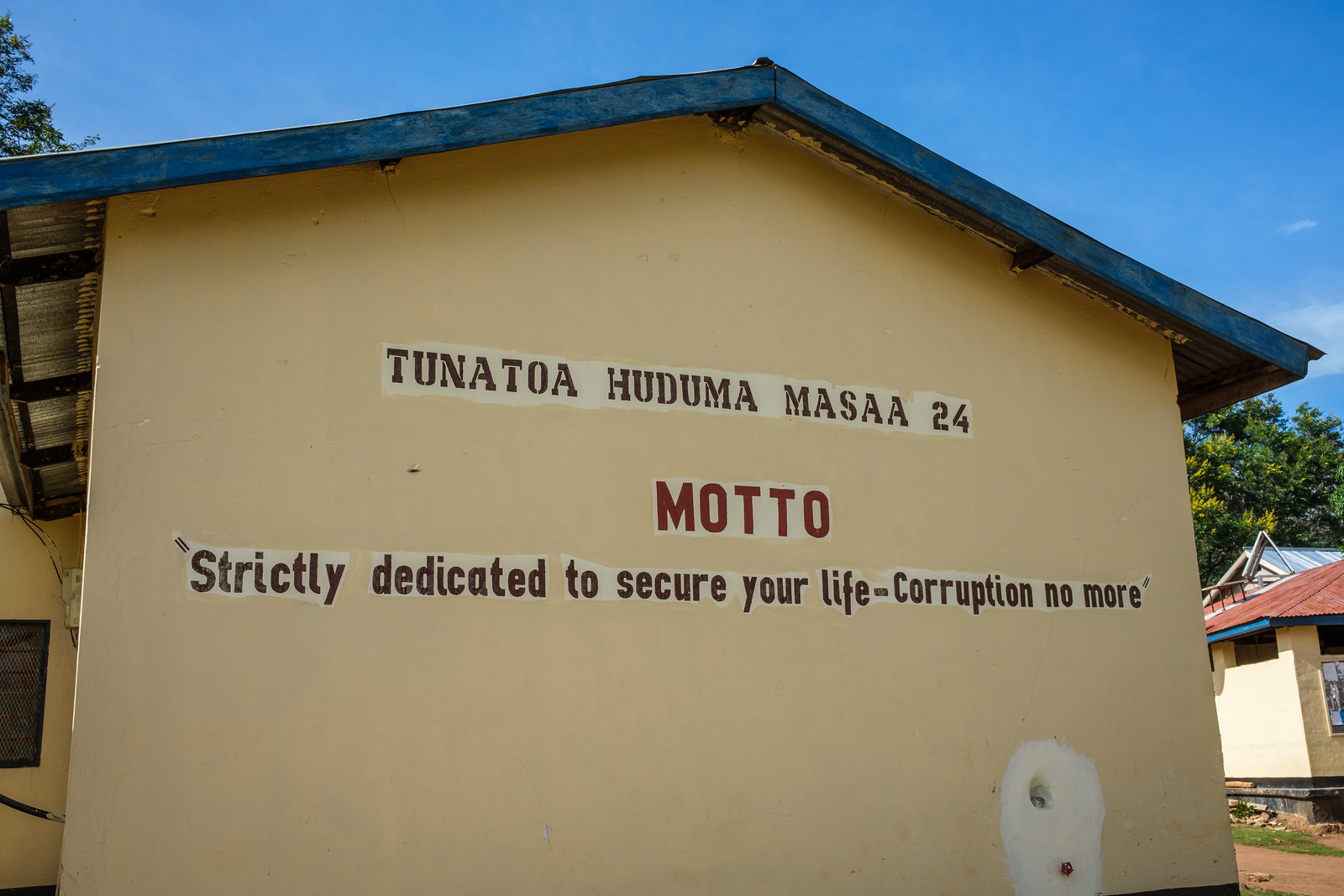This horizontal-rectangular image showcases the side of a somewhat worn beige stucco building with a peaked roof edged in blue trim. The wall prominently features text: the top line reads "Tuna Toa Huduma Masa'a 24," presumably the name or a significant phrase associated with the building. Below it, in large red letters, is the word "Motto," followed by a smaller black inscription: "Strictly dedicated to secure your life, corruption no more." Towards the bottom of the wall, there is a white section with visible pipes that may be part of a faucet control system. In the background to the right, there’s a smaller building with a similarly colored beige wall and blue-trimmed roof, although its roof's top is red. The image also contains elements of nature, with a tree to the middle right and some branches peeking out from the upper left corner. The sky in the background is clear and blue, adding contrast to the scene.